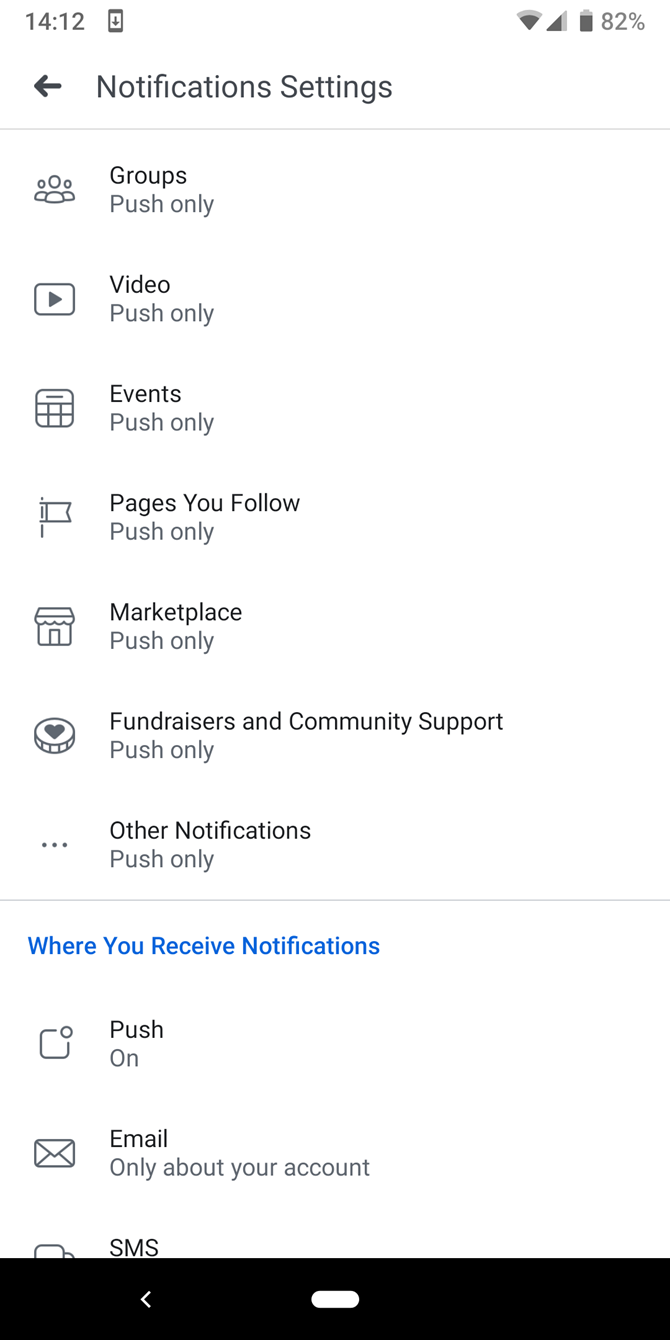A screenshot taken at 14:12 showing smartphone notifications and settings, with 82% battery life. The screen displays a list of notification categories, each accompanied by its respective icon: 
- "Groups," represented by three people, with "Push only" notification type. 
- "Video," indicated by a play button icon, also set to "Push only." 
- "Events," shown with a calendar icon, marked as "Push only."
- "Marketplace," featuring a market stand icon, listed as "Push only."
- "Fundraising and Community Support," with a heart icon, set to "Push only."
- "Other notifications," represented by three dots, configured to "Push only."

A section below these categories, highlighted in blue, indicates "Where you receive notifications," showing "Push" with its status as "On." Additionally, it specifies that email notifications are only for account-related updates. The screen also displays a section for SMS settings, and a black bar runs across the bottom of the screen.